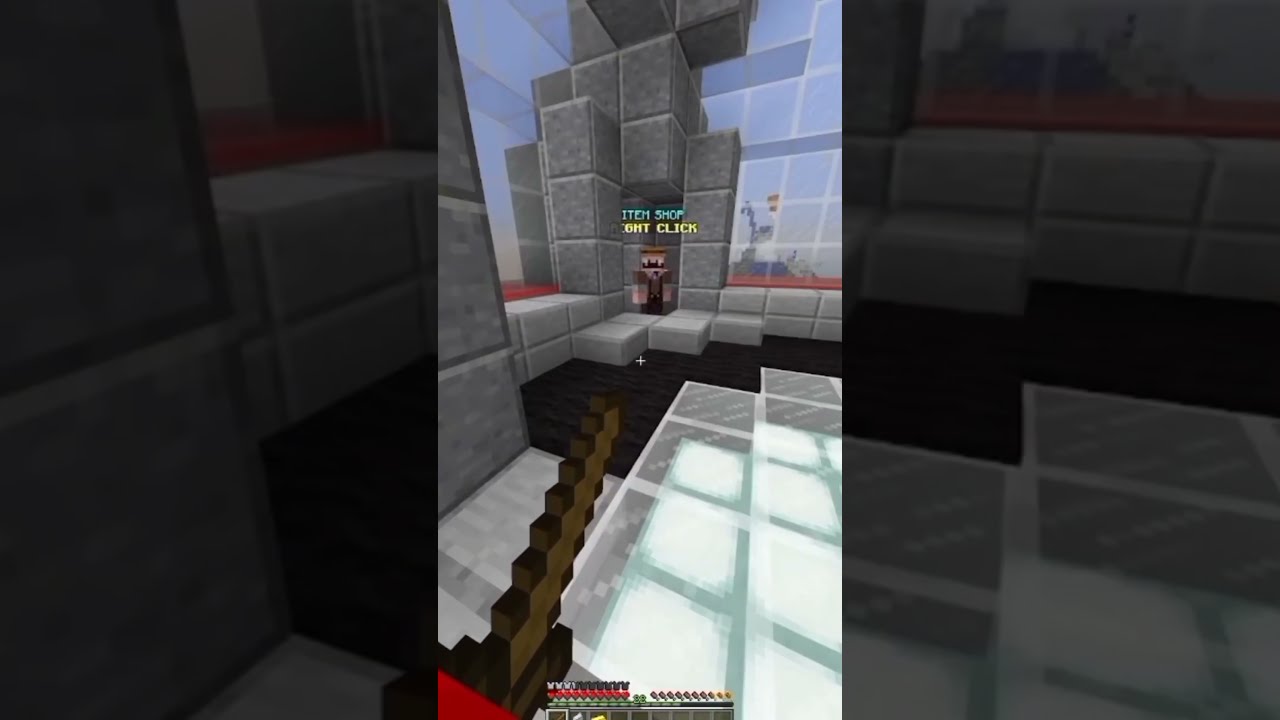The image appears to be a screenshot from the game Minecraft, characterized by its iconic blocky, 3D graphics reminiscent of an eight-bit aesthetic. Central to the image is a character, or avatar, equipped with a sword, standing on a floor that appears to be made of glass. The scene is set within a gray stone castle, containing towering cinder blocks and stacked gray blocks. Brown blocky stairs ascend to an elevated walkway in front of the character, who is facing towards us.

The avatar has a distinctly blocky form and features a large black mouth, wearing black overalls and a red shirt. Above the character, "Item Shop" is displayed in blue text, with an instruction that looks like "right click" in yellow. To the character's rear, more gray blocks and light blue windows can be seen ascending a wall. The image also contains UI elements typical of a video game, such as health icons, situated at the bottom of the screenshot. The left and right sides of the image feature darker, zoomed-in versions of the blocky castle environment.